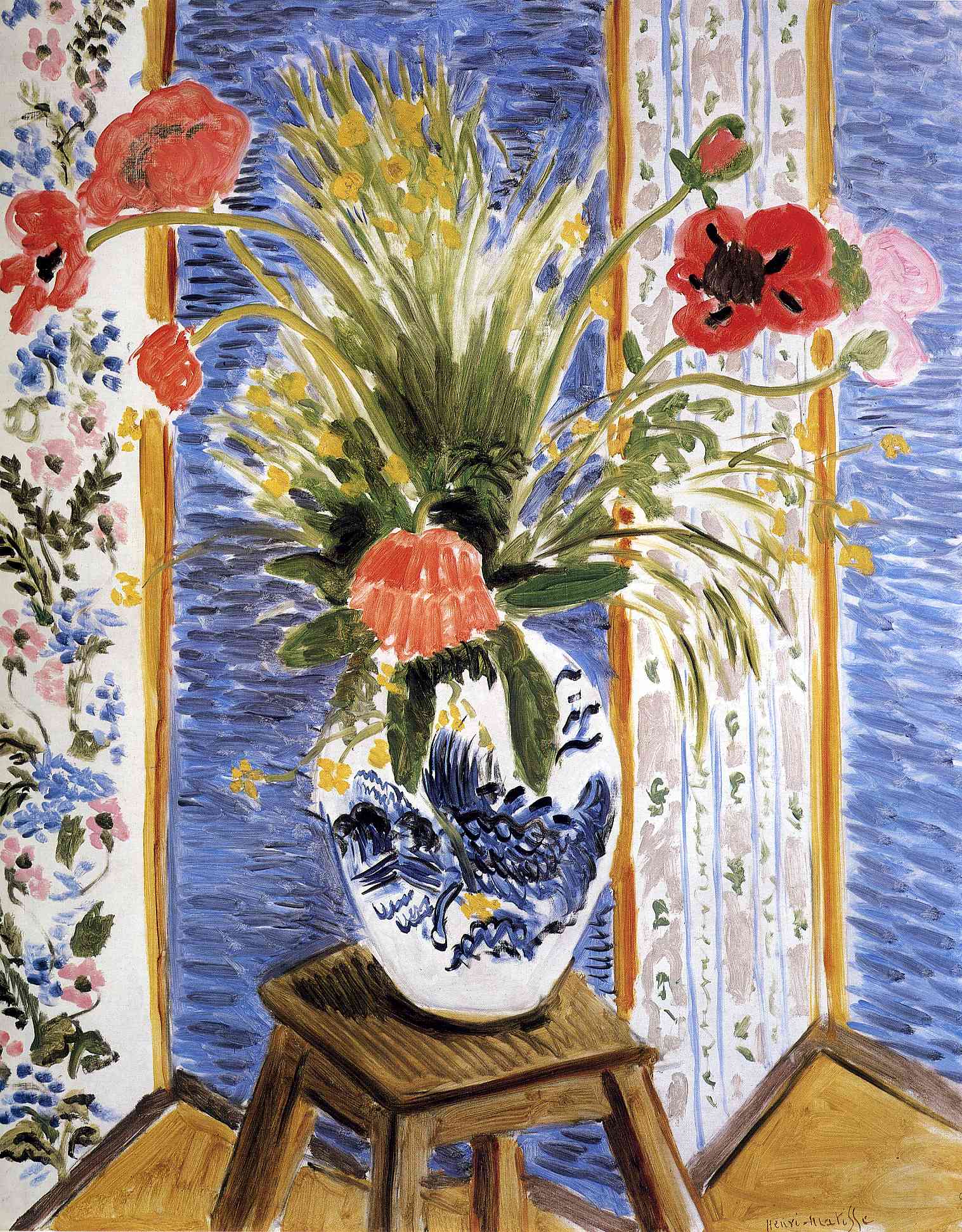This Impressionist-style watercolor painting captures a vivid indoor scene featuring a white vase adorned with blue and black decorative elements, possibly depicting mountains or a peacock, sitting on a dark brown, four-legged stool. The vase contains a striking arrangement of six to seven flowers, predominantly red with a few pink flowers, some fully bloomed while others are still opening. The flowers are complemented by small green plants and tiny yellow flowers, adding to the vibrant display. The background showcases a folding screen with four panels: one adorned with pink and blue flowers, another with stripes and floral patterns, and two painted in solid blue. The setting includes a light brown hardwood floor and additional dark brown wood trim. The scene is framed by a wall displaying sections of bright blue and floral wallpaper, featuring pink, blue, and green hues, creating a rich and colorful backdrop without any text or figures present, underscoring the serene and detailed composition of the space.